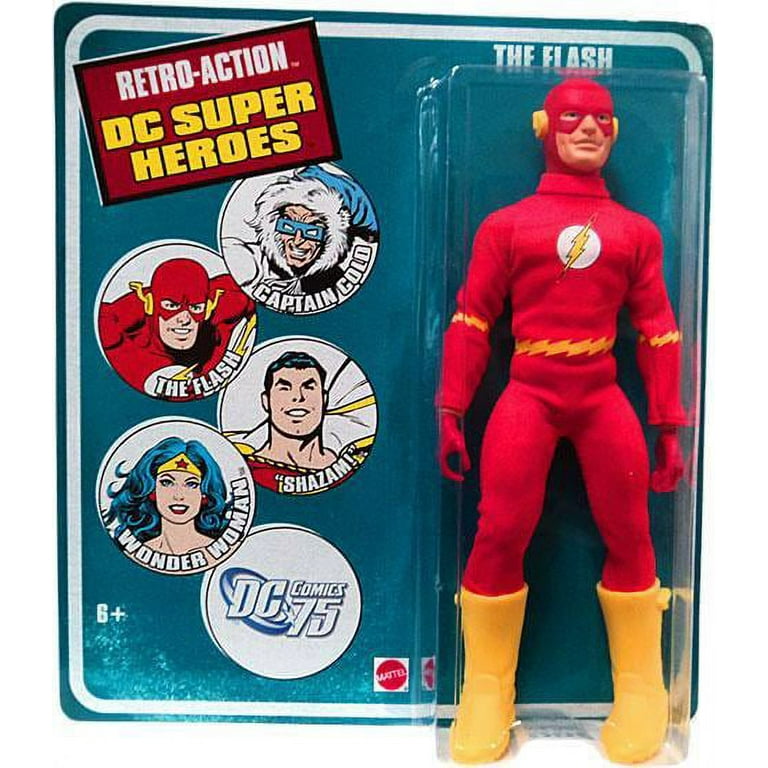This is a detailed photograph of a vintage action figure of the superhero, The Flash, still in its original packaging. The Flash figure stands prominently on the right side of the packaging encased in a clear hard plastic bubble, protecting the figure itself, which features a red outfit with bright yellow boots and yellow lightning bolts at the waist and elbows. The Flash's chest sports his iconic emblem: a white circle with a yellow lightning bolt. His face is partially masked, with the lower half exposed and yellow lightning accents over his ears.

The action figure is attached to a rectangular blue cardboard backboard with a white border. The branding at the top of the packaging features "The Flash" in white font. On the left side of the packaging, a red rectangle with white text reads "Retro-Action," followed by "DC Super Heroes" in yellow lettering. Surrounding these words are colorful circles showcasing the heads of other action figures from the collection: Captain Cold in a blue coat, another depiction of The Flash, Shazam, and Wonder Woman. Additionally, a red circle at the bottom mentions the manufacturer, Mattel, while the bottom left corner denotes an age recommendation of "6+". A notable detail is the "DC Comics 75" logo, indicating this collectible toy is part of a special anniversary edition. These nostalgic details and the inclusion of multiple images of other characters suggest the toy may date back to as early as the 1950s.